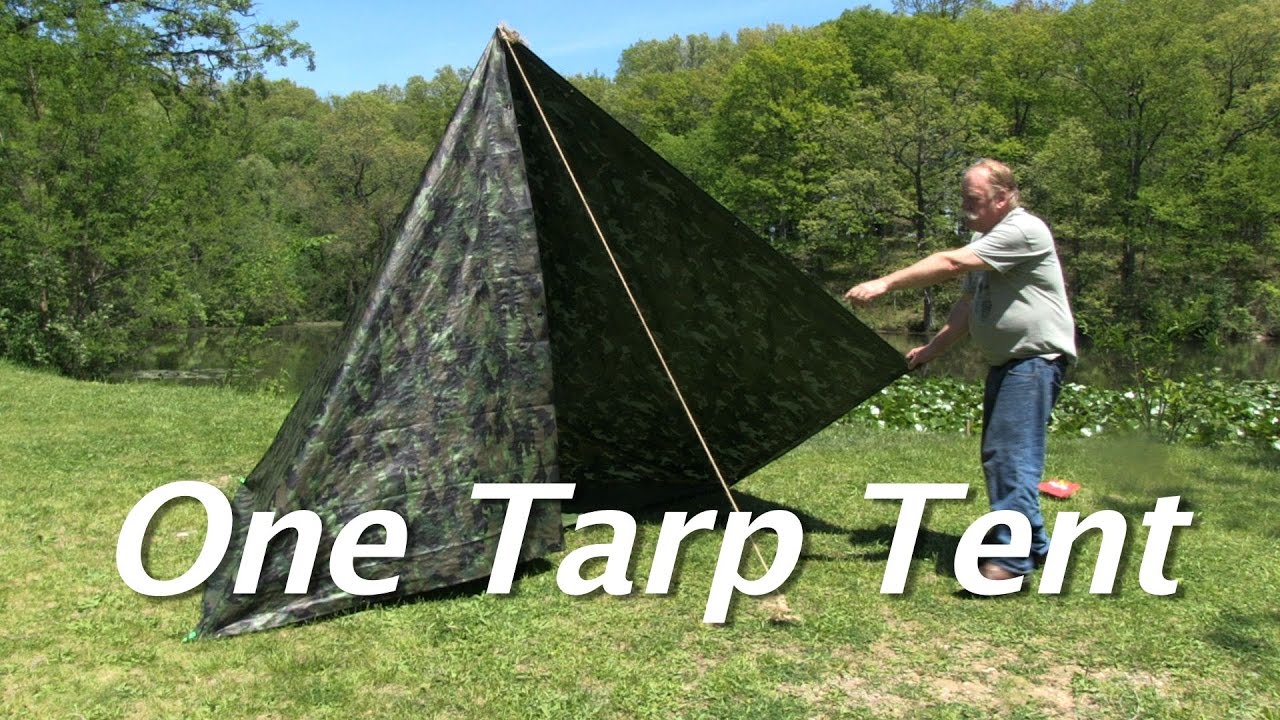In a verdant natural setting, a photograph captures an older, slightly overweight man with a whitish mustache erecting a tent made from a dark camouflage tarp. The man, wearing a light green t-shirt and baggy blue jeans, stands on the right side of the image, holding a corner of the tarp in his left hand while his right hand points towards something within the tent. The tarp, a dark green and black color with lighter green flecks, is pitched into a triangular shape, with a thin, light-colored rope securing its peak to the ground. The backdrop reveals tall, lush green trees and a hint of a small creek or pond. At the bottom of the image in large, three-dimensional white letters, the caption reads "One Tarp Tent." A red object lies on the grass nearby, adding a touch of contrast to the scene.